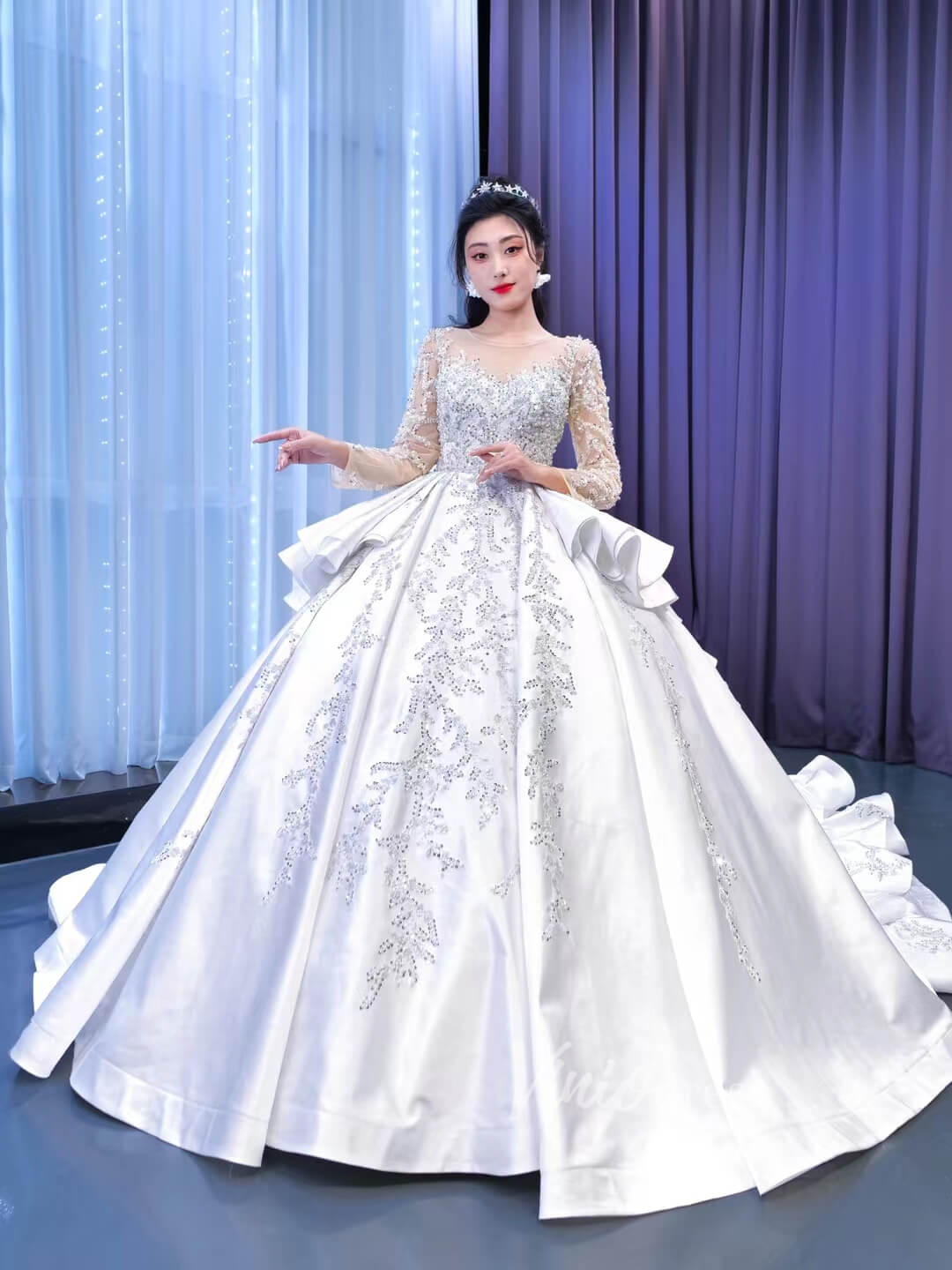This is a photograph of a young Asian woman, possibly Japanese, standing on a gray floor and posing in front of two curtains—a light blue sheer curtain to the left and a purple stage curtain to the right. She is wearing a very elaborate, fairytale-like wedding gown that exudes the elegance of a ballroom-style dress, reminiscent of Cinderella. The gown features a sheer upper section adorned with jewels and crystals, and its voluminous skirt, constructed with hoops, expands into a bell shape, creating a dramatic and imposing silhouette that includes a trailing train.

Her dark black hair is complemented by a tiara with silver stars, and she accessorizes with large diamond-like earrings. She wears striking red lipstick. The gown is made of white silk and includes intricate embroidery, possibly resembling leaves, on both the front and the sheer bodice. Her hands are positioned in an unusual manner: one is held in front of her midriff while the other extends to her side, with her arms bent at the elbows. She stands directly in the center of the image, gazing right at the camera.